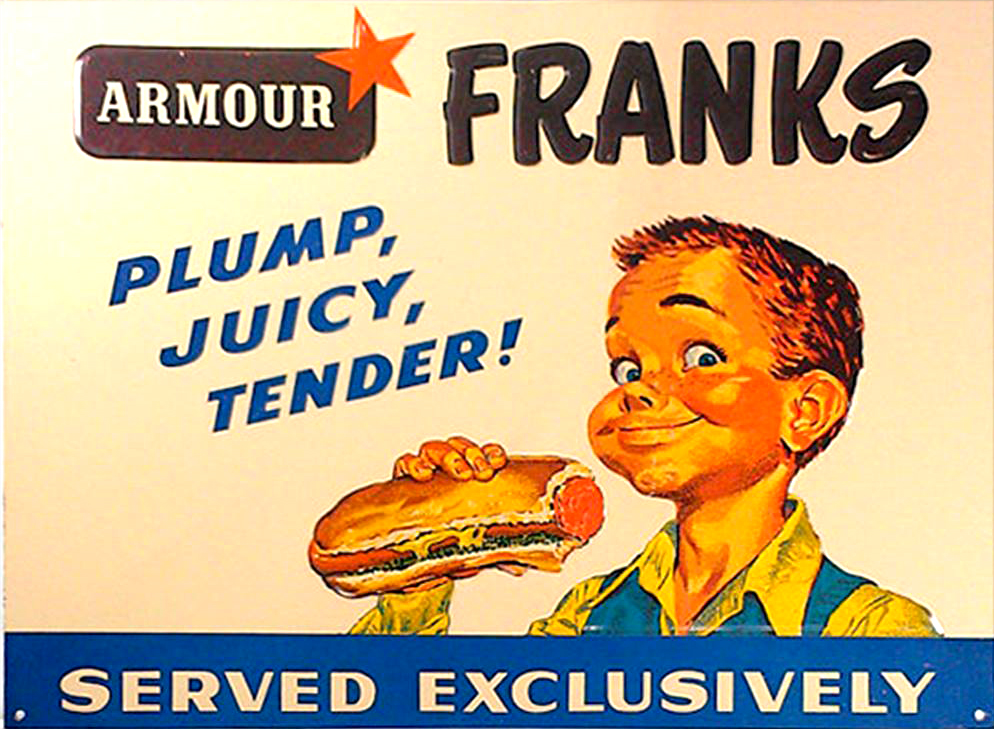The image is a vintage advertisement for Armor Franks, arranged horizontally. It features a lightly toned background that transitions from a salmon color on the left to a slightly darker shade on the right. In the top left corner, a brown curved rectangle bears the word "ARMOR" in white uppercase letters, accompanied by an orange star on its upper right. To the right of this, "FRANKS" is displayed in bold, black, uppercase letters. Below, the words "PLUMP, JUICY, TENDER!" are stacked vertically in blue, uppercase letters. 

To the right, there is a cheerful illustration of a young boy with short, spiky, orangish-brown hair and wide blue eyes. His cheeks are stuffed, and he sports a closed-mouth smile while holding a large hot dog with a bite missing. The boy wears a yellow shirt with a blue collar and vest. At the bottom of the ad, a blue banner reads "SERVED EXCLUSIVELY" in white, uppercase letters, bordered by a red stripe.